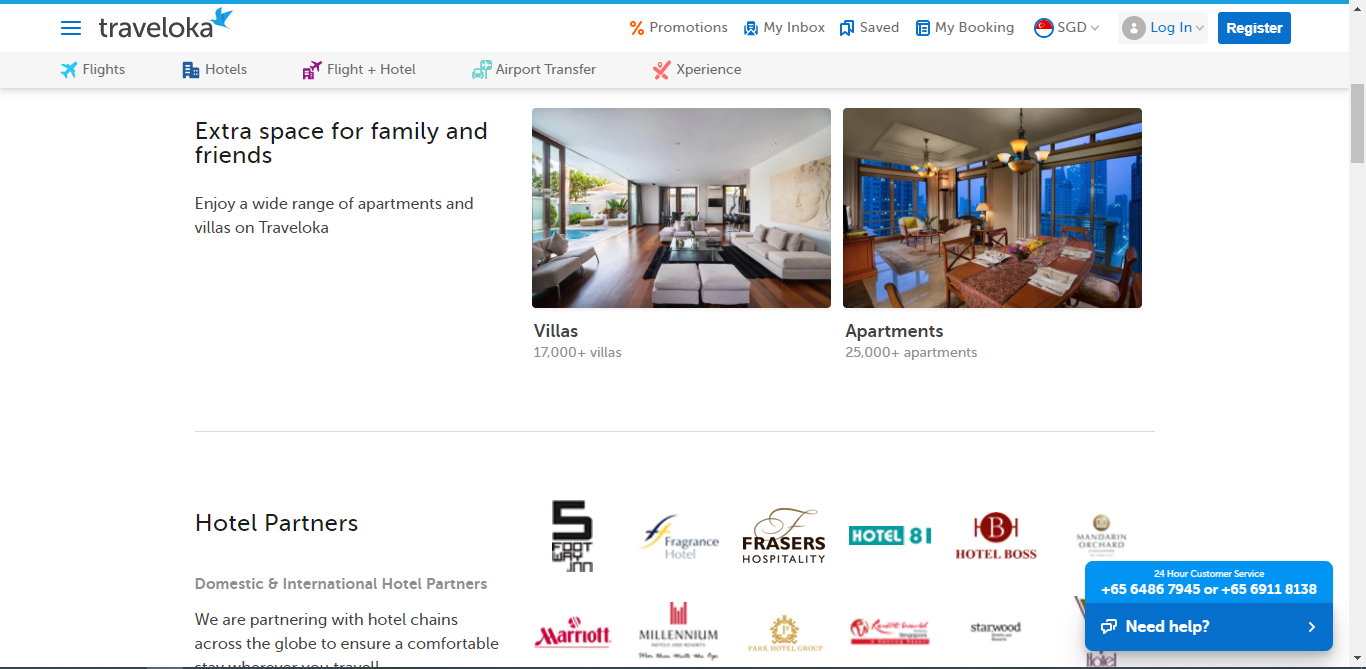A screenshot of a travel booking website named Trapalotka. The page is predominantly white with a horizontal blue stripe running across it. The main menu options displayed at the top of the page include Flights, Hotels, Flights and Hotels, Airport Transfer, Promotions, My Inbox, Save, My Booking, Login, and Register. Highlighted in the center of the page are Trapalotka's extensive accommodations: over 17,000 villas and over 25,000 apartments. The site also showcases partnerships with various prominent hotel chains such as Marriott, Millennium, Dominic and International Hotel Partners, Fraser's Hospitality, and Hotel Boss. A helpful feature for users is a small blue box with white text labeled "Need Help." A blue stripe at the top of the screen completes the streamlined aesthetic.